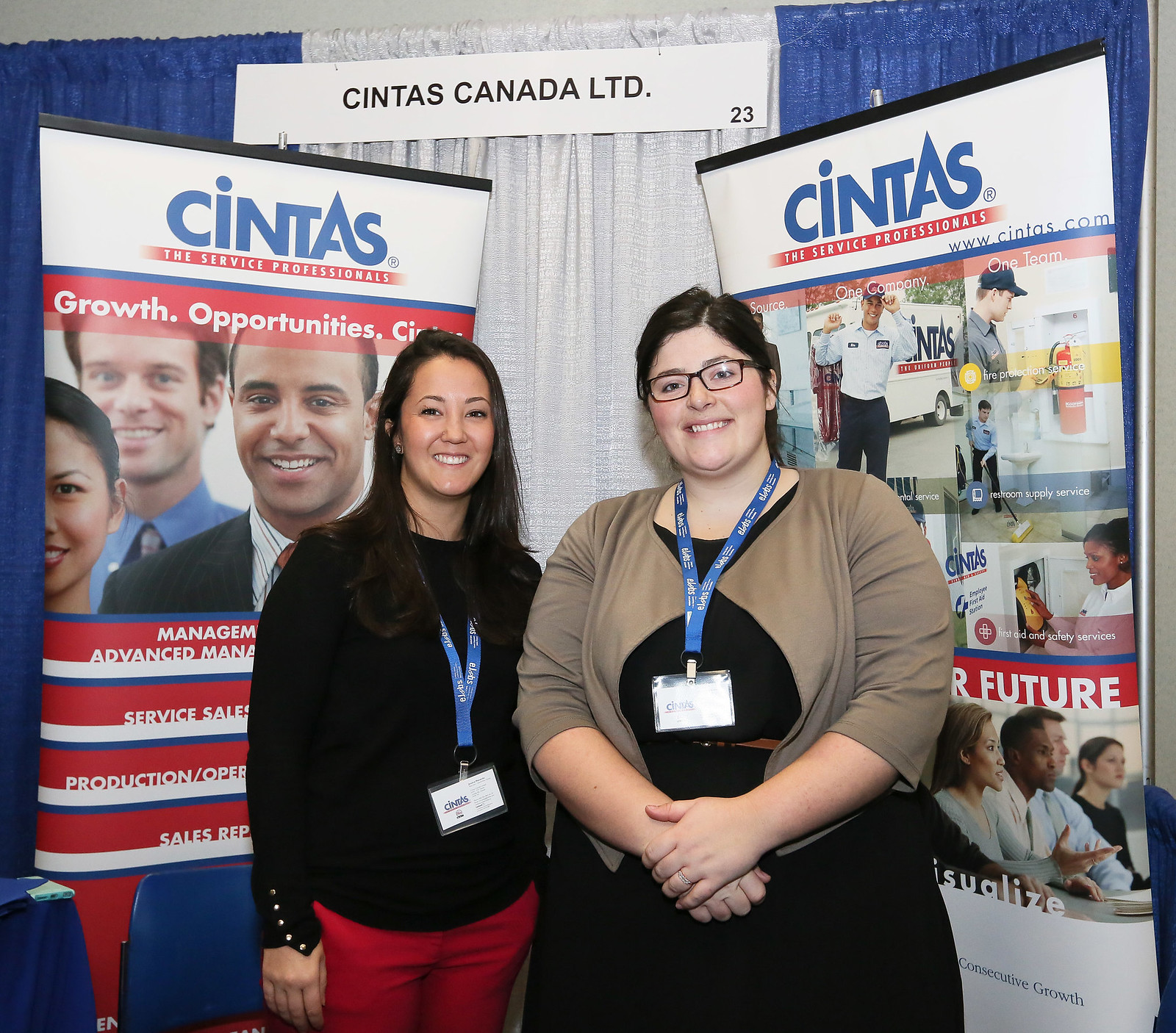The image, taken indoors at a convention, features a blue and white backdrop with a paper sign at the top that reads "Cintas Canada LTD." Surrounding the two women in the foreground are two large banners. The banner on the left displays a picture of several smiling individuals with the text "Cintas, the service professionals, Growth Opportunity" in white font on a red bar. Below this, albeit partially obscured, are words like "management," "advanced service sales," and "production." The banner on the right includes images of people engaged in various professional activities, such as driving a truck, making a phone call, and participating in a meeting. 

In between these banners stand two women who appear to be employees of Cintas, identifiable by the company IDs on their blue lanyards. The woman on the left has long dark hair, wears a black top, and red pants, while the woman on the right, with short dark hair and glasses, is dressed in a black dress and a brown vest.